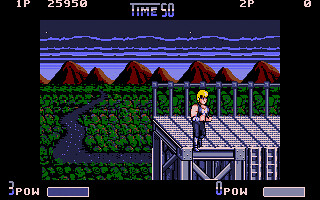In this image from a video game, the scene is framed by a black border, with the text "Time 50" displayed prominently at the top in gray lettering. A white streak cuts across this text, adding a sense of urgency or action. The background depicts a night-time setting with dark skies, under which a serene landscape unfolds. Distant, shadowy mountains stand tall, with what appears to be a vast sea lying at their base.

In the foreground, a gray trail meanders through a dense forest, leading to a flat, sleek steel platform reminiscent of aluminum bleachers. On this platform stands a muscular character with blonde hair, clad in black pants. The character gazes out into the landscape, seemingly pondering the vast expanse before them. Additional game HUD elements include "POW 0" and "POW 3", indicating various game statistics. This image encapsulates a moment of pause and reflection within the game's immersive environment.